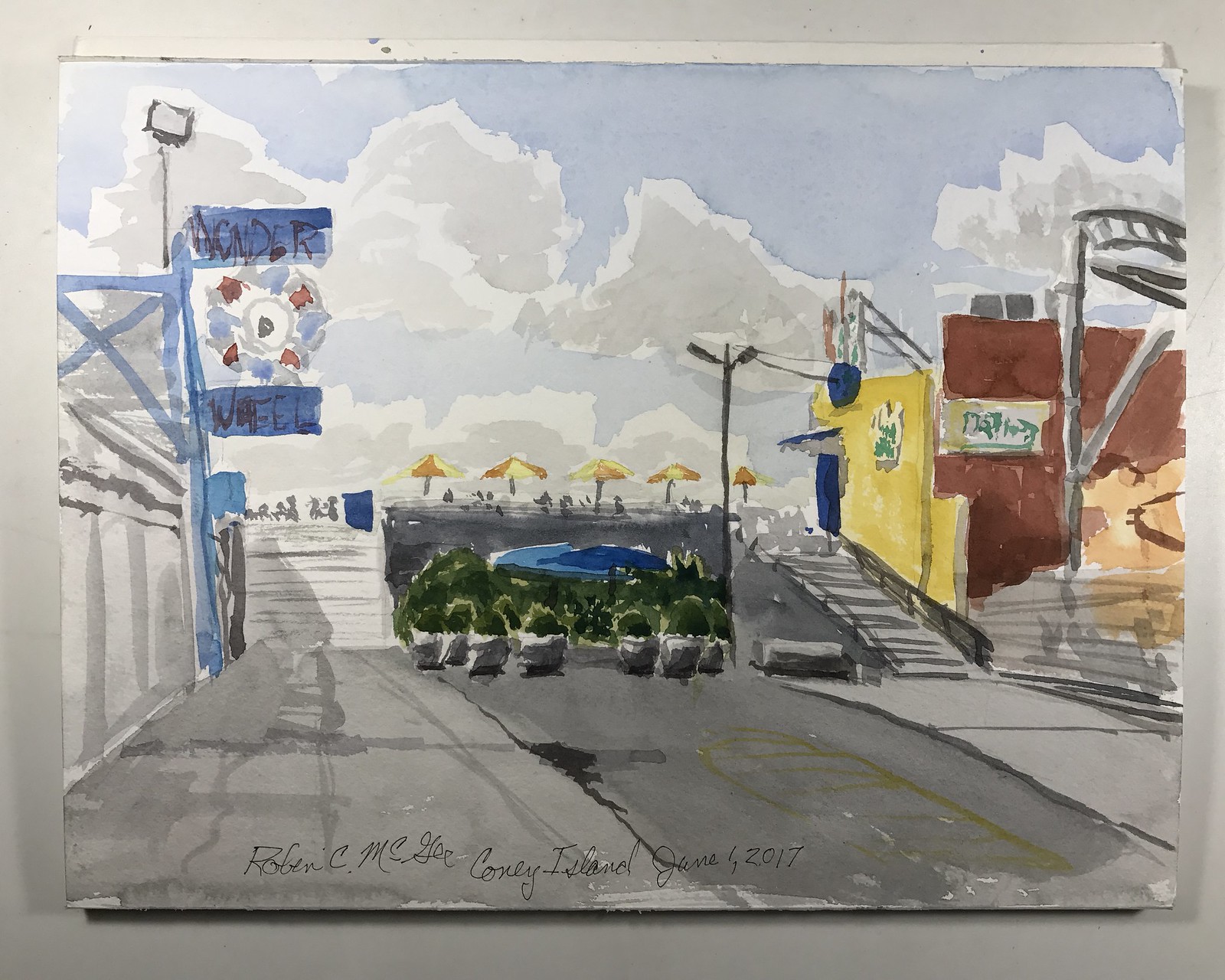This image features a watercolor painting of Coney Island, signed by Robin C. McGee and dated June 1st, 2017. Against a black background, the painting predominantly uses gray tones, especially for the roadway and sky, which also includes blue hues and some gray clouds. On the left-hand side, there's a sign that reads "Wonder Wheel" in blue with black lettering, depicting a Ferris wheel with blue and brown dots between the words. Below the sign, there are green plants painted along the bottom edge. Towards the middle ground, there is a blue lake or pool with five triangular yellow and orange umbrellas above it. The right-hand side of the painting features a brown building next to a yellow one, with some indiscernible signs on their facades. A gray staircase rises in front of these buildings. Despite the loose and muddy watercolor style, the painting captures the essence of a bustling wharf or city street scene, characterized by various colorful elements and architectural details.